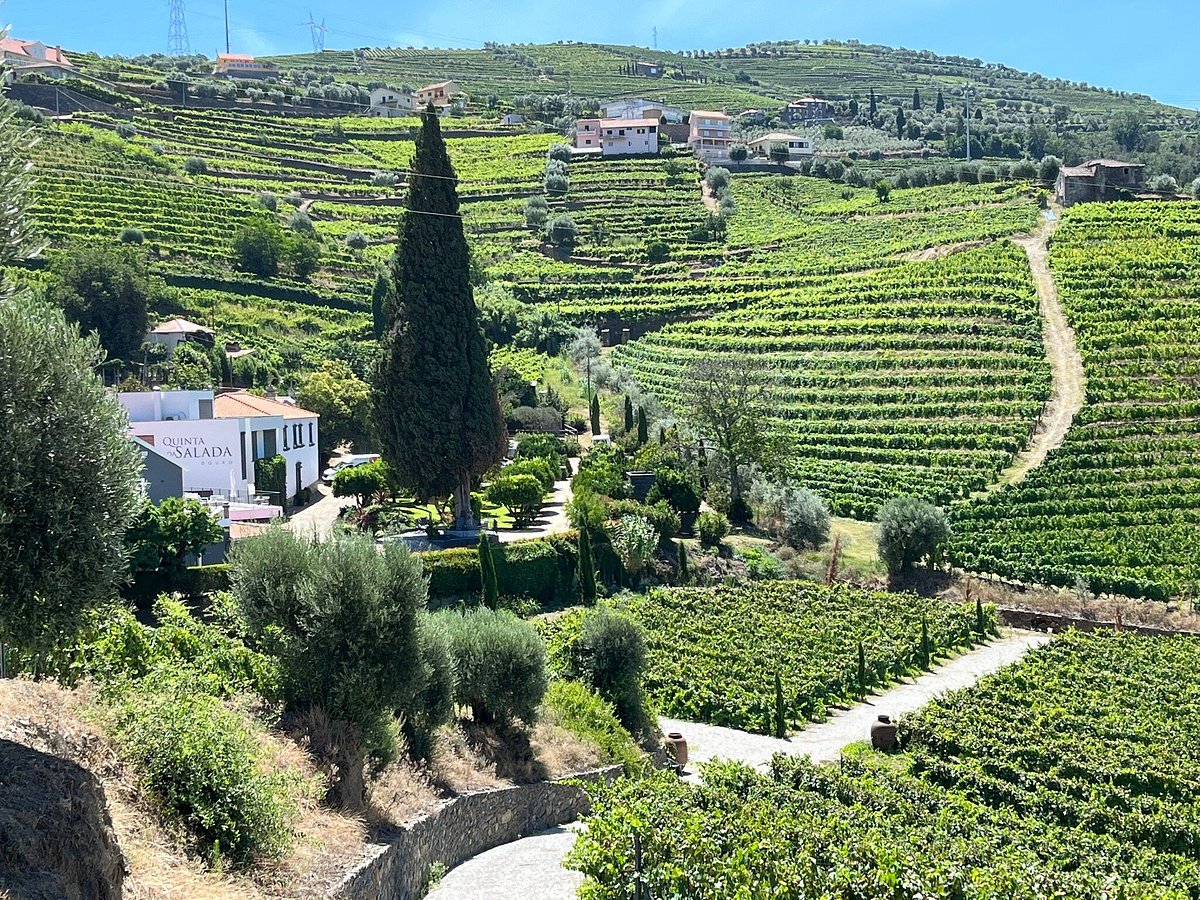This is a color photograph of a sunny, hilly agricultural scene, capturing the essence of a terraced vineyard, possibly located in Italy. The focus is primarily on the rolling hillsides, meticulously divided into sections for growing what appear to be wine grapes. Scattered across the landscape are several low, sturdy trees and tall shrubs, adding a touch of greenery to the otherwise orderly vines.

In the foreground and stretching up towards the mid-ground, small dirt roads zigzag through the terraced fields, guiding the eye up the hills. Prominently, a white building with large, clear lettering that reads "Quinta Salata" sits on one of these hills, suggesting perhaps the name of the vineyard. Nearby, additional paths and dirt roads trace their way up the hillside, enhancing the structured beauty of the landscape.

Dotted across the upper slopes of the hills are various houses and buildings, characterized by their traditional red-tiled roofs. These homes add a touch of rustic charm while indicating the human presence and agricultural activity in the area. In the farthest reaches of the scene, a stone wall and electrical transmission towers are faintly visible, indicating the edge of this cultivated terrain.

The sky above is a bright, clear blue, with a hint of morning fog blending softly along the horizon, giving a serene backdrop to this pastoral tableau. This well-detailed image captures both the natural beauty and the agrarian diligence of a picturesque vineyard.